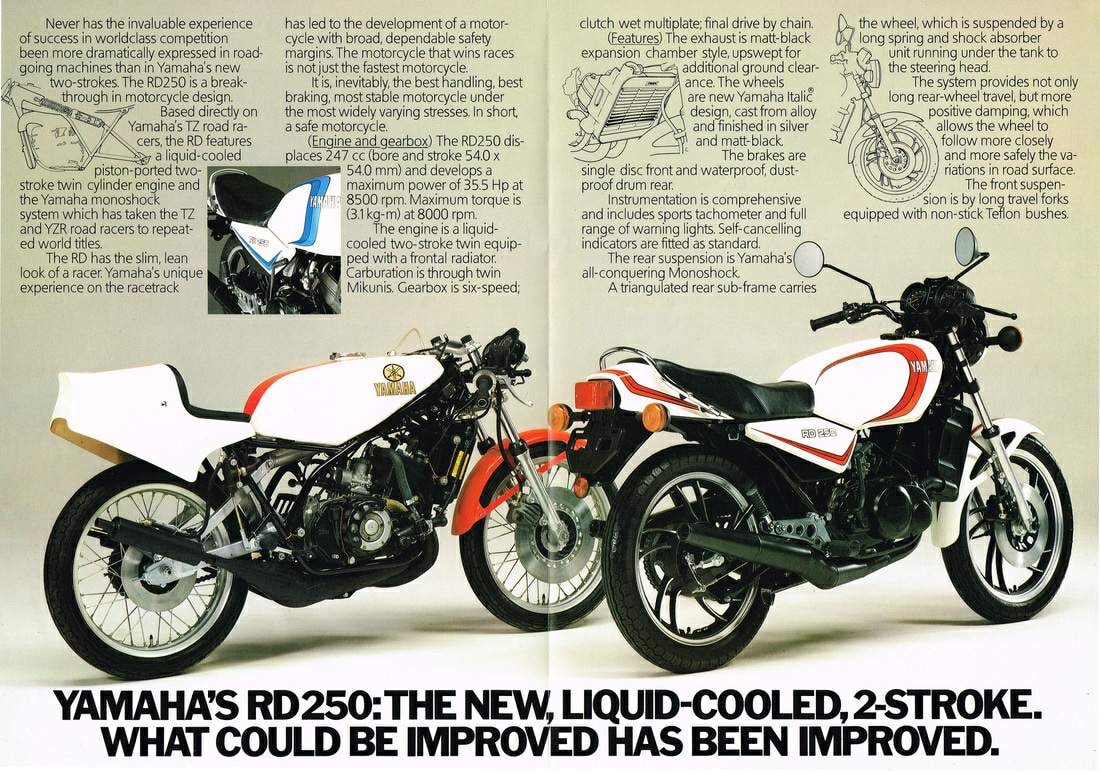The image is an advertisement that resembles a folded brochure, evident from a crease running down the center. The spread showcases Yamaha's RD250 motorcycles, featuring a studio setting with a white background. Both motorcycles are white with orange-red and white accents, facing sideways to the right. The motorcycle on the left has an orange front rim, while the one on the right has a white front rim. Each page of the brochure has detailed paragraphs describing the motorcycles, with two paragraphs on each side discussing the new features and improvements. 

Above the left motorcycle, there’s a small inset image showing the rear end of another blue and white Yamaha motorcycle. The substantial text at the bottom of the spread reads: "Yamaha's RD250: The new liquid-cooled two-stroke. What could be improved has been improved." 

The upper half of the image elaborates on the technical advancements and features of the RD250, stating: "Never has the invaluable experience of success in world-class competition been more dramatically expressed in road-going machines than in Yamaha's new two-strokes. The RD250 is a breakthrough in motorcycle design, based directly on Yamaha's TZ Road Racers. The RD features a liquid-cooled, piston-ported, two-stroke, twin-cylinder engine and the Yamaha Monoshock system, which has taken the TZ and YZR Road Racers to repeated world titles." 

Alongside the text, there are smaller illustrations and diagrams highlighting the enhancements in the engine, gearbox, exhaust system, and other components. The advertisement merges technical details with visual appeal to emphasize the RD250's advanced engineering and superior design.